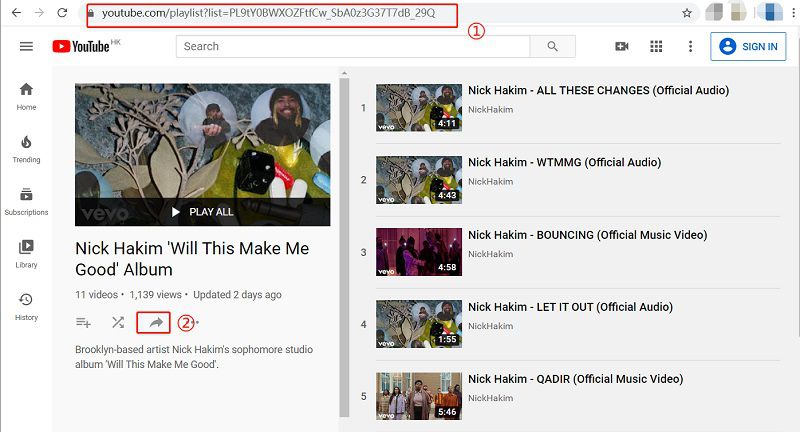The image is a screenshot of a YouTube desktop interface, highlighting a specific playlist page. At the top, inside a red rectangular box, the URL in the search bar reads: "youtube.com/playlist?list=PL9TY0BWXOFZFTFCW_SBA0Z3G37T7DB_29Q". Below the search bar, the YouTube logo is prominently displayed, featuring the company name and the iconic red play button to its left. To the left of the logo is the settings button, depicted as three stacked horizontal lines. Sequentially arranged below this are the links for Home, Trending, Subscriptions, Library, and History.

Beneath the top navigation, the main content of the page showcases a playlist titled "Nick Hakim - Will This Make Me Good (Album)". This playlist contains a total of 11 videos and has garnered 1,139 views. The page indicates that the playlist was last updated two days ago. Below the playlist title, there's a "Play All" button, facilitating the continuous playback of all videos in the playlist.